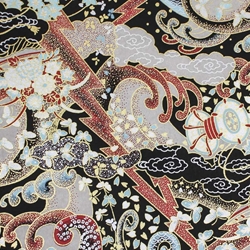This captivating piece exudes the essence of modern nouveau art, reminiscent of intricate tablecloth designs, wall art, or even ornate wallpapers. The composition hinges on a striking lightning bolt motif that diagonally slices through the artwork from the upper left to the lower right. Its red exterior frames a blend of purplish-brown hues, standing bold against the dark blue and grainy brown undertones that pervade the background.

Interspersed throughout are an array of dynamic elements—flower petals and blossoms meld with abstract butterflies, curls, and swerves, creating an impression of elegant realism. To the right, an enigmatic form emerges, evoking imagery of a light bulb, an alien figure, or possibly a vessel. The left side teems with curlicues, additional petals, and sprinkled dots, all intertwined within tentacle-like formations, further enhancing the piece's intricate design.

Gold squiggly lines and white shapes punctuate the upper left-hand corner, adding to the tapestry-like quality of the image. The vivid palette includes bursts of red, blue, and purple, contributing to a visually busy tapestry that evokes the richness of Victorian style and the decorative flair found in casino rugs or traditional carpet designs. The overall effect mimics a festive explosion of swirling forms and vibrant colors within a cohesive, modern artistic impression on a dark, textured background.